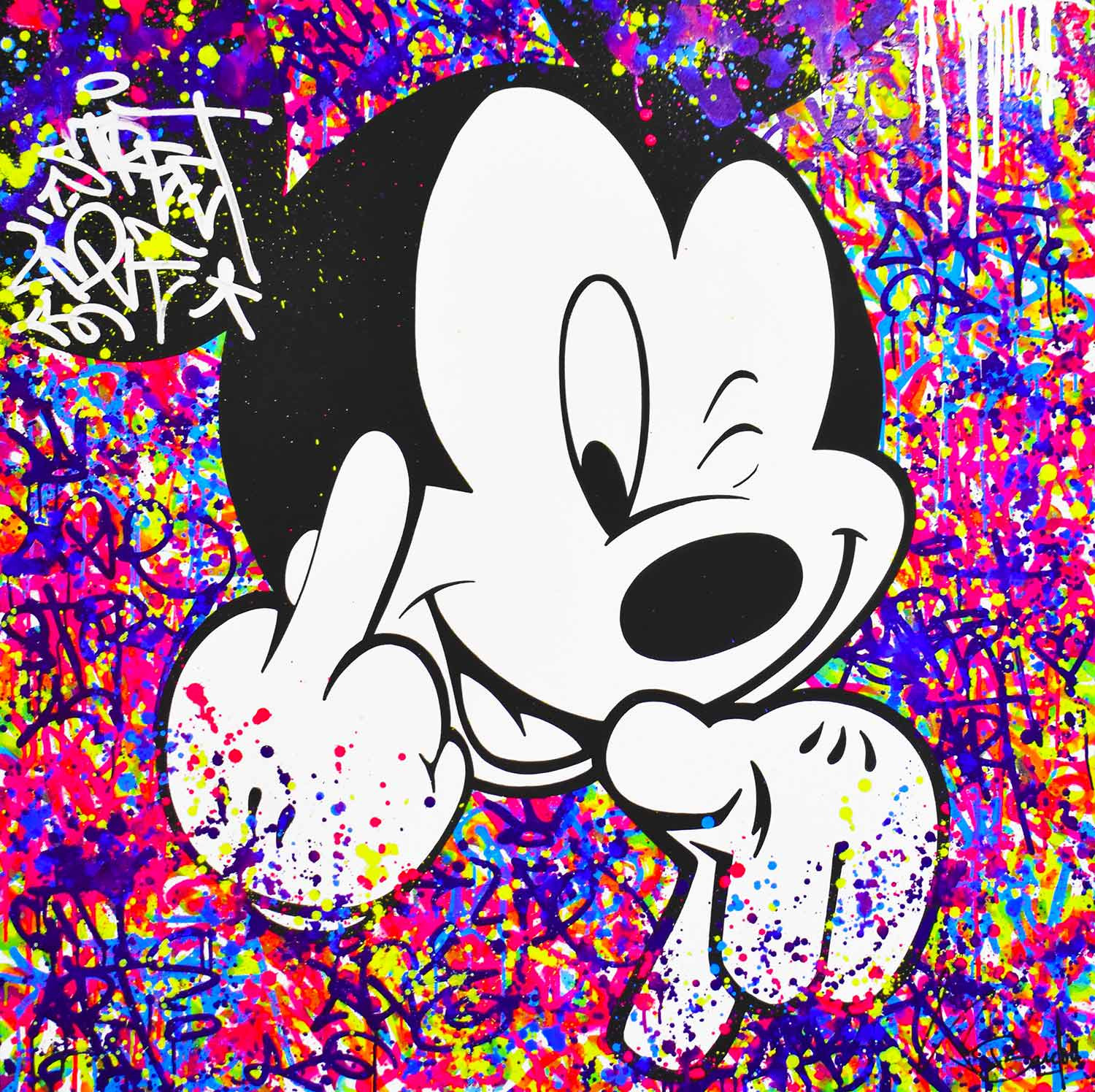The image depicts Mickey Mouse winking and smiling, with his left eye open and his right eye closed. He sports his classic white gloves, with one hand pointing towards the viewer while the other hand makes an obscene gesture. His nose is a black oval, horizontally aligned across his face. Surrounding Mickey are vibrant splotches of paint in a variety of colors, including blue, red, yellow, pink, purple, and white, resembling confetti. Additionally, graffiti-like scribbles and writing, mostly illegible, are scattered throughout the background, adding a chaotic yet colorful atmosphere to the composition. Some of these graffiti elements also appear on his white glove in the upper left corner of the image.